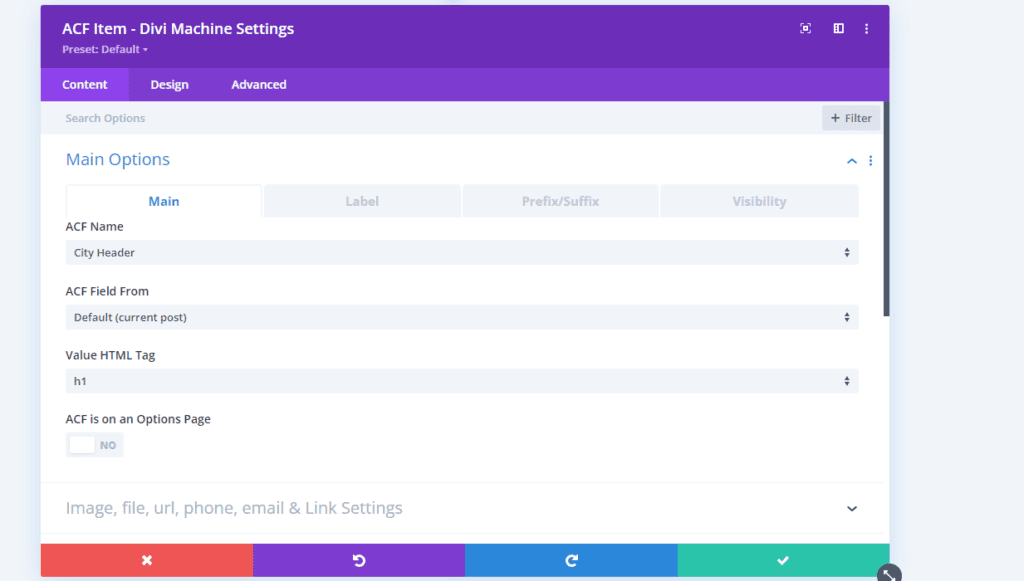The image displays an open page with a predominantly purple background at the top. At the very top, text reads, "ACF Item, Give Image Setting, Preset Default." Below this, there are several tabs labeled "Content," "Design," and "Advanced," with "Content" being currently selected. 

Within the "Content" tab, header text declares "Search Options," followed by a section named "Main Option," which is highlighted in blue. Here, there are additional tabs titled "Main," "Labeled," "Prefix or Suffix," and "Visibility," with "Main" having been chosen, indicated by its blue color while the others remain grey.

The first input field is labeled "ACF Name: City Header," accompanied by a dropdown menu that allows the selection of various components. The second field is labeled "ACF Field: From," offering options such as "Default" and "Current Post," which reveals further choices when clicked. The third input field is titled "Value: HTML Tag" and features a dropdown menu set to "H1," providing other HTML tag options upon interaction.

Below these fields, it states "AFC is on an option page," with a toggle switch currently set to "No," which can be toggled to "Yes" if desired. At the bottom of the section, there's a dropdown menu for "Image, File, URL, Font, Image and Link Setting" allowing for further selection.

At the very bottom of the page, there are four distinct buttons: a white "X" on a red background (likely for closing or canceling), a purple button labeled "Preview," a blue button labeled "Load," and a green button featuring a check mark (possibly for saving or accepting changes).